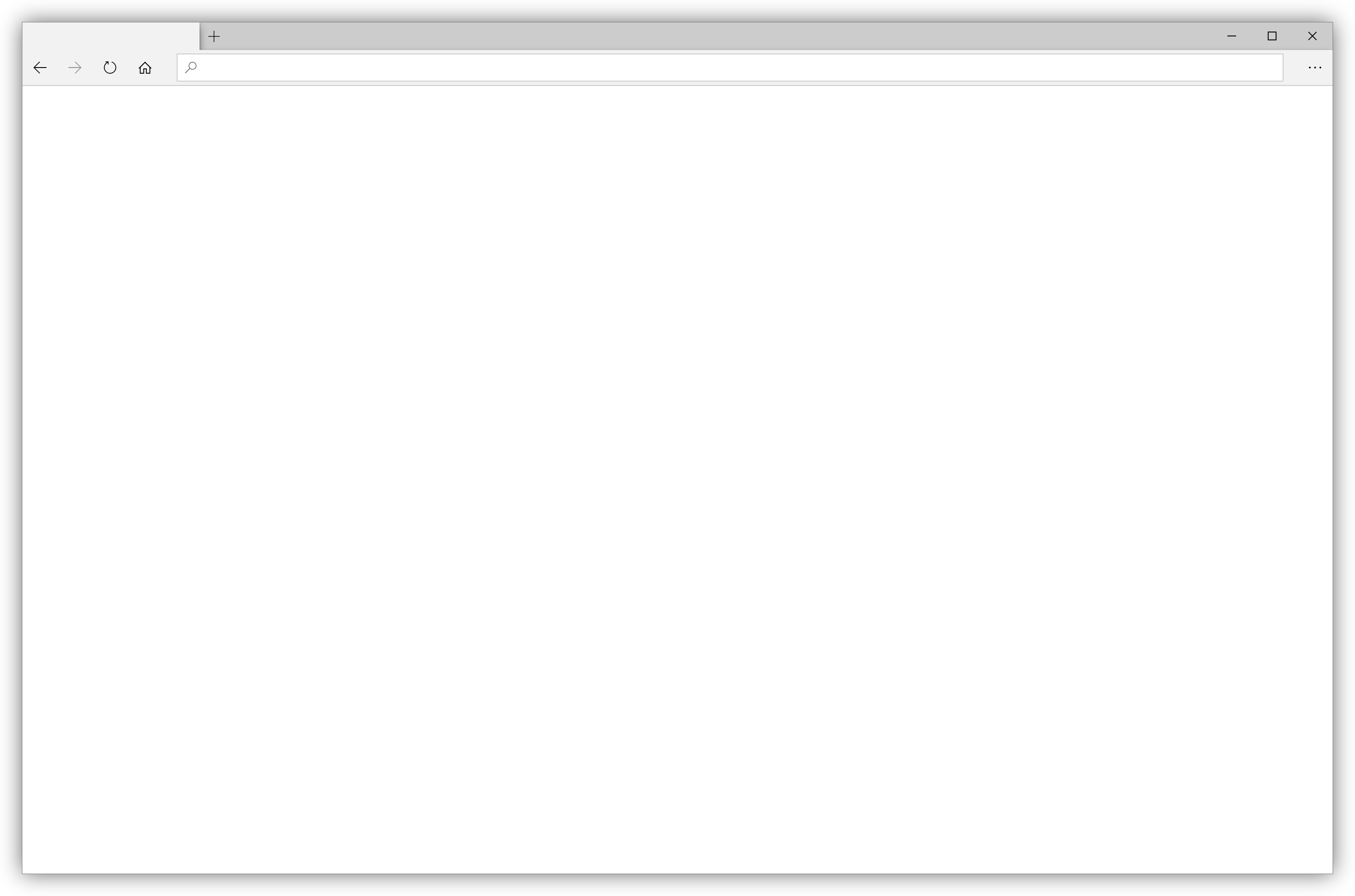This screenshot showcases a desktop browser interface with its default elements visible, though the main page is entirely blank and white. The browser’s header features a light gray section on the left, transitioning to a dark gray across the top. Centered prominently within this header is a large search bar. 

On the far left bottom corner of the header’s light gray section, there are navigation icons: a back arrow, a forward arrow, a refresh icon, and a home icon. At the top left corner, within the same light gray area, there's a plus sign to open a new tab. 

Contrastingly, the top right corner of the header's dark gray section contains window control buttons: minimize, maximize, and close (X). The white of the blank page starkly highlights these elements.

Surrounding all four edges of the screenshot is a subtle light gray shading, creating a lifted, three-dimensional effect as though the image is hovering above the background.